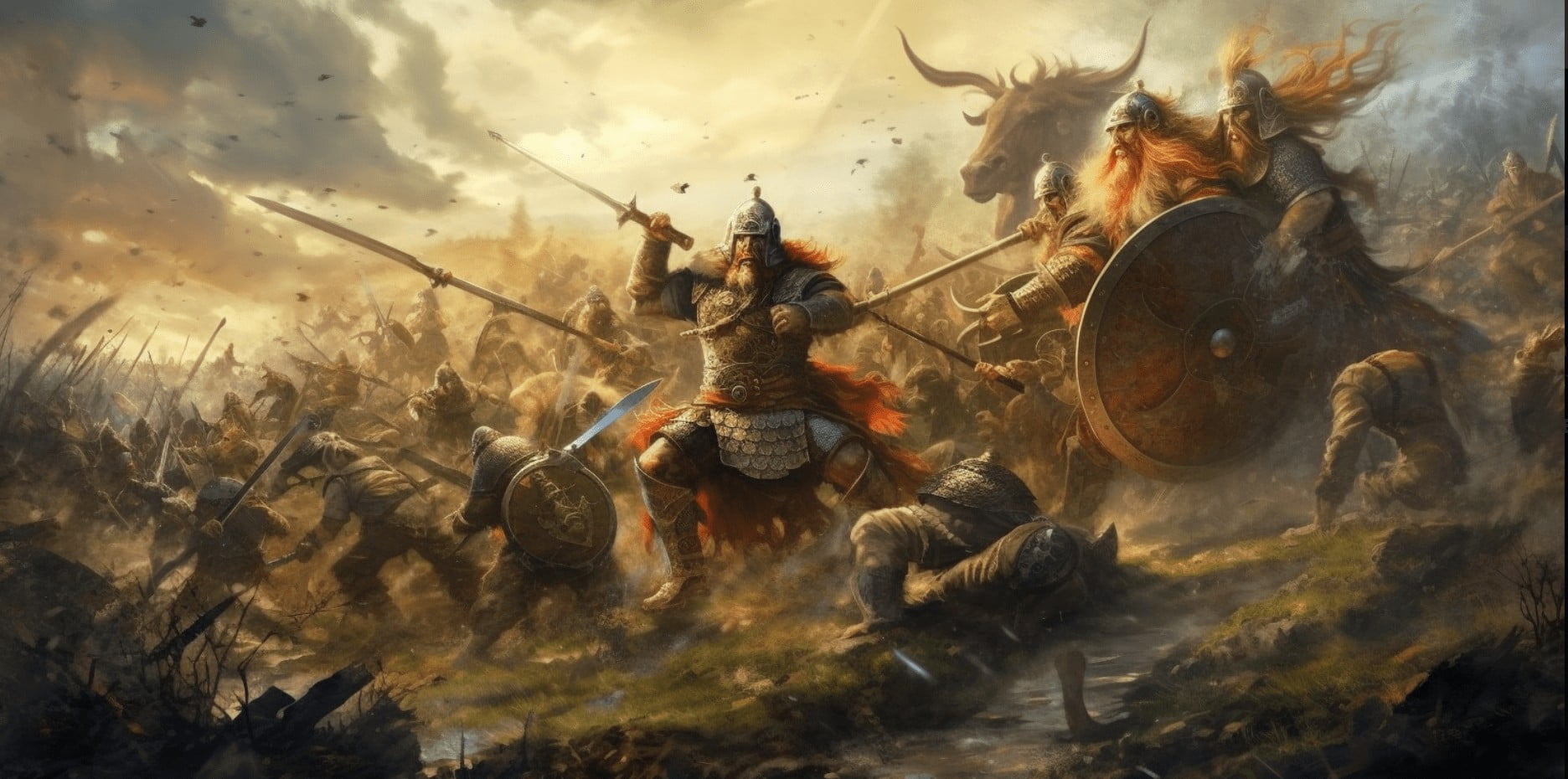The image is a vivid and chaotic battle scene, potentially computer-generated or painted in a rectangular format. The sky above is filled with dense clouds or smoke, with sunlight trying to break through, illuminating the action below. Dominating the battlefield are several giants clad in armor, their long red hair and beards flowing dramatically. One giant at the center of the image brandishes a sword or spear in one hand, poised to strike, with his other hand raised as if ready to punch. 

Behind him and slightly off-center to the right towers a massive brown bull with imposing horns, overseeing the chaotic fray. Another giant with a shield and also with long red hair stands close by. To the left of the central giant is a much smaller soldier who barely reaches the giant's chest, highlighting the immense size difference. 

The battlefield itself is a mix of muted brown and green hues, scattered with rocks and possibly segments of a fence towards the bottom left. Further, to the right and below the bull's head, men in silver helmets are gathered, some seemingly positioned behind a large wheeled vehicle. These men, along with the giants, are part of a larger force clashing with enemies both up and down the slopes of the terrain. The scene is imbued with a sense of frantic movement and impending violence, capturing the intensity and turmoil of the battlefield.